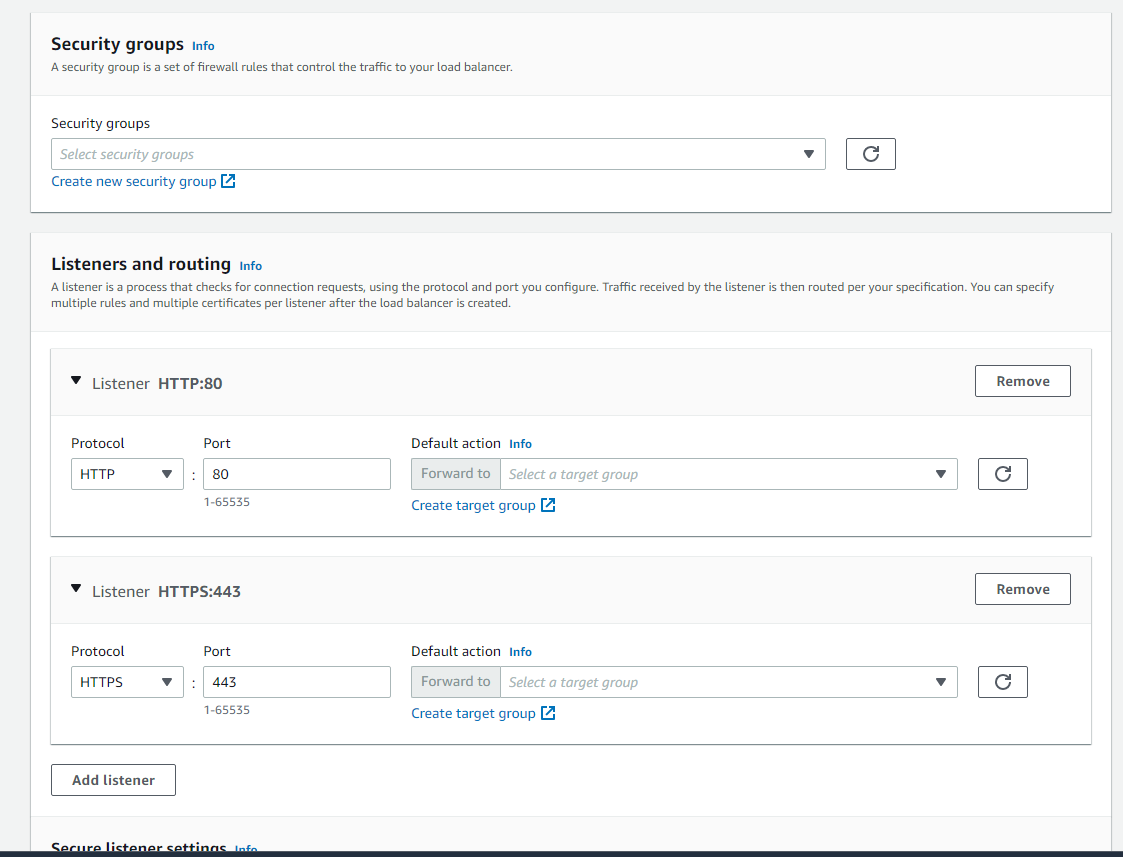A screenshot displays a webpage open on a computer, showcasing a clean, minimalistic design with a light gray background adorned with various informational boxes. At the top, a section titled "Security Groups" provides a detailed explanation: "Security groups setup firewall rules that control the traffic to your load balancer." Below, an actionable button labeled "Create New Security Group" invites user interaction.

Directly underneath, another section labeled "Listeners and Routing" offers insights: "A listener is a process that checks connection requests using the protocol and port you configure. Traffic received by the listener is then routed according to your specifications, allowing for multiple rules and certificates per listener." Further down, two pre-configured listeners are highlighted: "Listener HTTP 80" and "Listener HTTPS 443," with an option to add additional listeners if needed.

The overall layout is straightforward and user-friendly, designed with simplicity in mind.